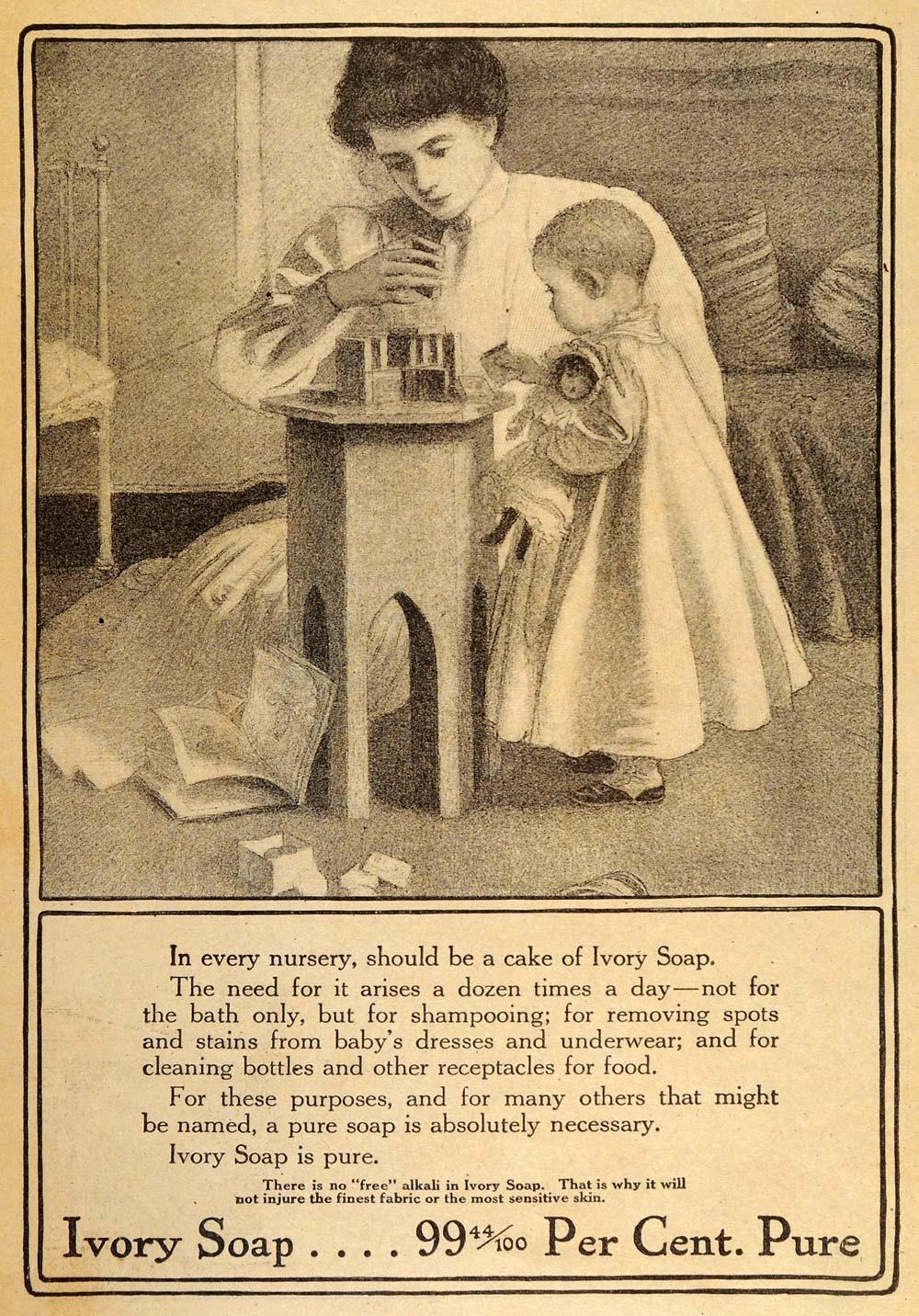In this vintage advertisement, the aged paper carries a yellowed tint, indicating its historical origin. The black illustration prominently features a young mother dressed in early 1900s attire, wearing a long-sleeved white dress with a collared neckline. She stands poised in front of a small table adorned with building blocks. To the right, a little girl, also in period clothing, holds a doll close to her chest and faces the table. The child has very short hair and wears a long-sleeved dress that reaches her ankles. The text beneath the illustration reads: “In every nursery should be a cake of Ivory Soap. The need for it arises a dozen times a day, not for the bath only, but for shampooing, for removing spots and stains from baby's dresses.” Finally, at the bottom of the advertisement, bold text proclaims: “Ivory Soap, 99 and 44/100 percent pure.”